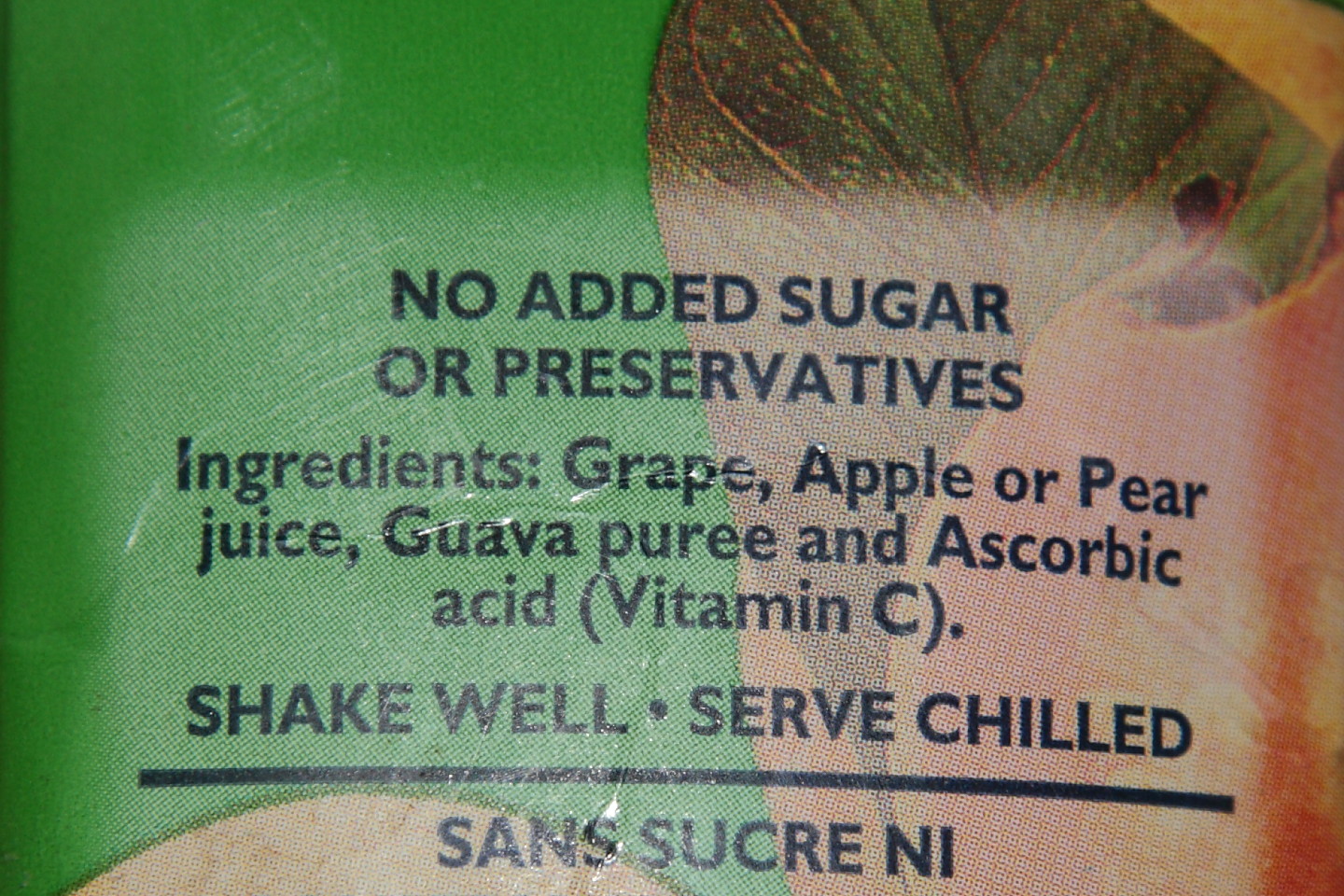A high-resolution close-up image showcases the label on a juice bottle or carton. The label features a vibrant design with a prominent green leaf and a piece of fruit in orange and yellow hues, set against a kelly green background. Prominently displayed in bold black print are the words "No Added Sugar or Preservatives." Below this, in smaller black font, the list of ingredients includes grape juice, apple or pear juice, guava puree, and ascorbic acid (Vitamin C). Further down, in larger, capital letters, the instructions "SHAKE WELL" are followed by a small dot and the phrase "SERVE CHILLED." A black line is drawn beneath these instructions, separating them from additional text, which appears to be in French.